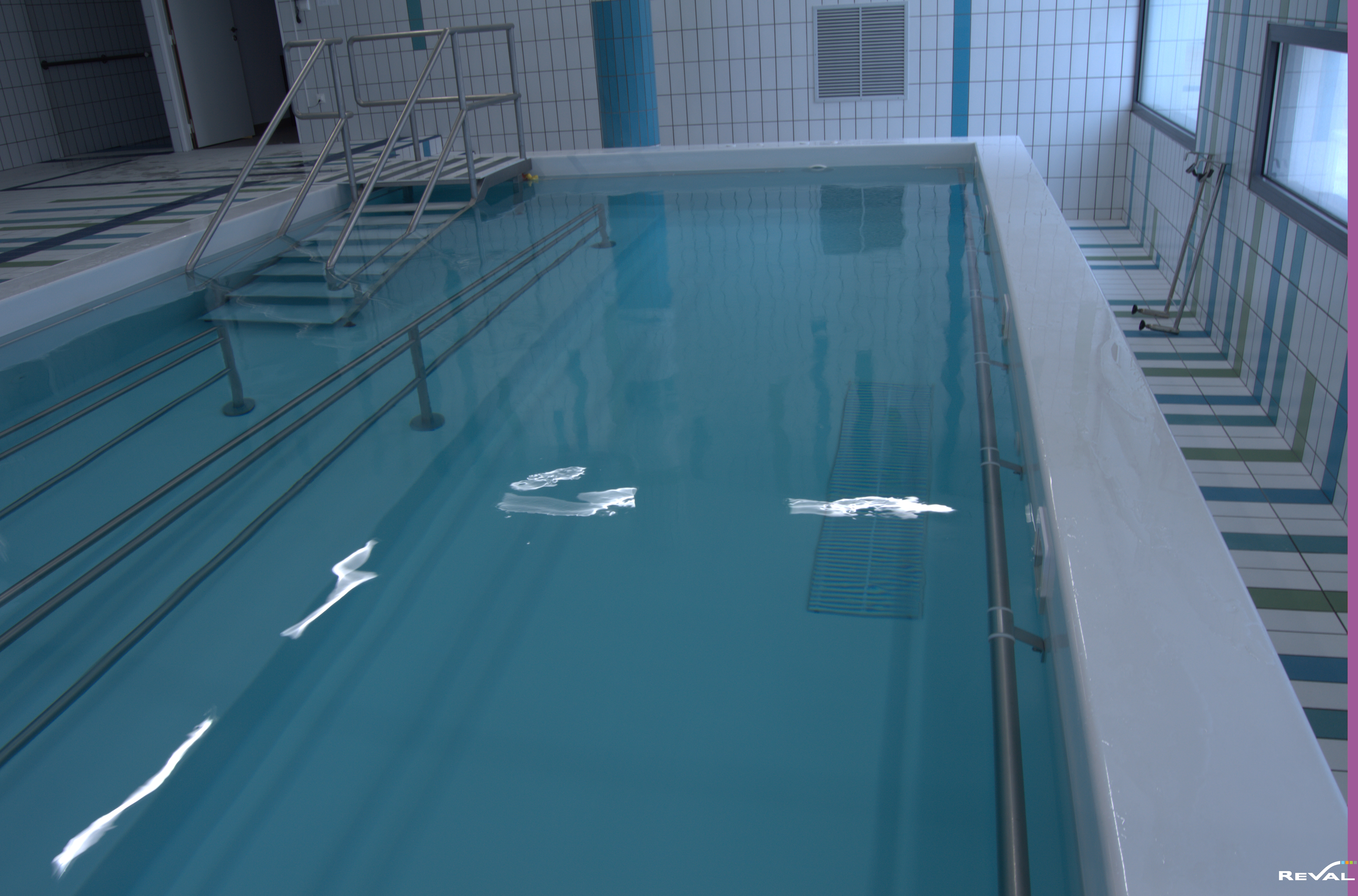The image depicts an indoor swimming pool situated predominantly on the left side of the photo. The waters of the pool are pristinely clear, revealing four white substances within, moving diagonally from the bottom left to the middle right of the pool. The pool features a silver stairway with banister railings in the top left corner. Adjacent to the pool, the interior includes walls tiled in white, blue, and green hues, with some sections appearing predominantly white. The space around the pool is accentuated by metallic rods and poles, adding to the room's structure. On the right side of the image, there are two windows, and further right, an open doorway is visible. The tile flooring underscores a clean and orderly environment with a marble-like appearance. Notably, the word "REVAL" can be seen inscribed in the bottom left corner of the picture.